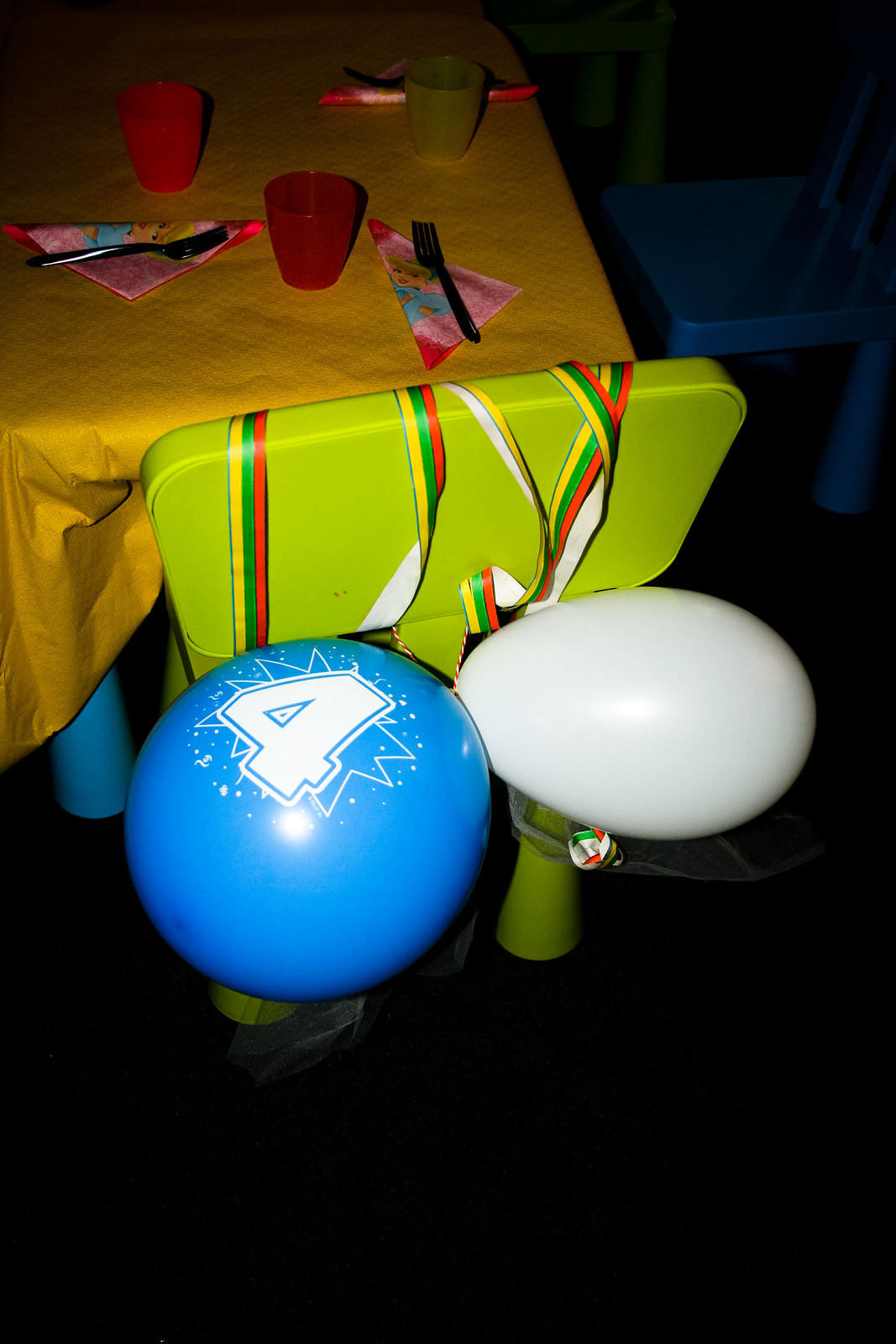In this dimly lit photograph, the camera's flash highlights a festive birthday party setup. A blue table with blue legs sits in the upper left corner, adorned with a golden yellow tablecloth. On the table are several plastic cups in red, yellow, and green, and napkins in pink, blue, and red, each accompanied by a plastic fork. A blue chair is partly visible in the upper right corner, while a neon green children’s chair with colorful straps—yellow, green, and red—occupies the center, connected to two balloons. One balloon is nearly deflated and white, while the other is blue with the number four written in white. The dark surroundings obscure additional details, focusing attention on the brightly colored objects that prepare for the celebration.